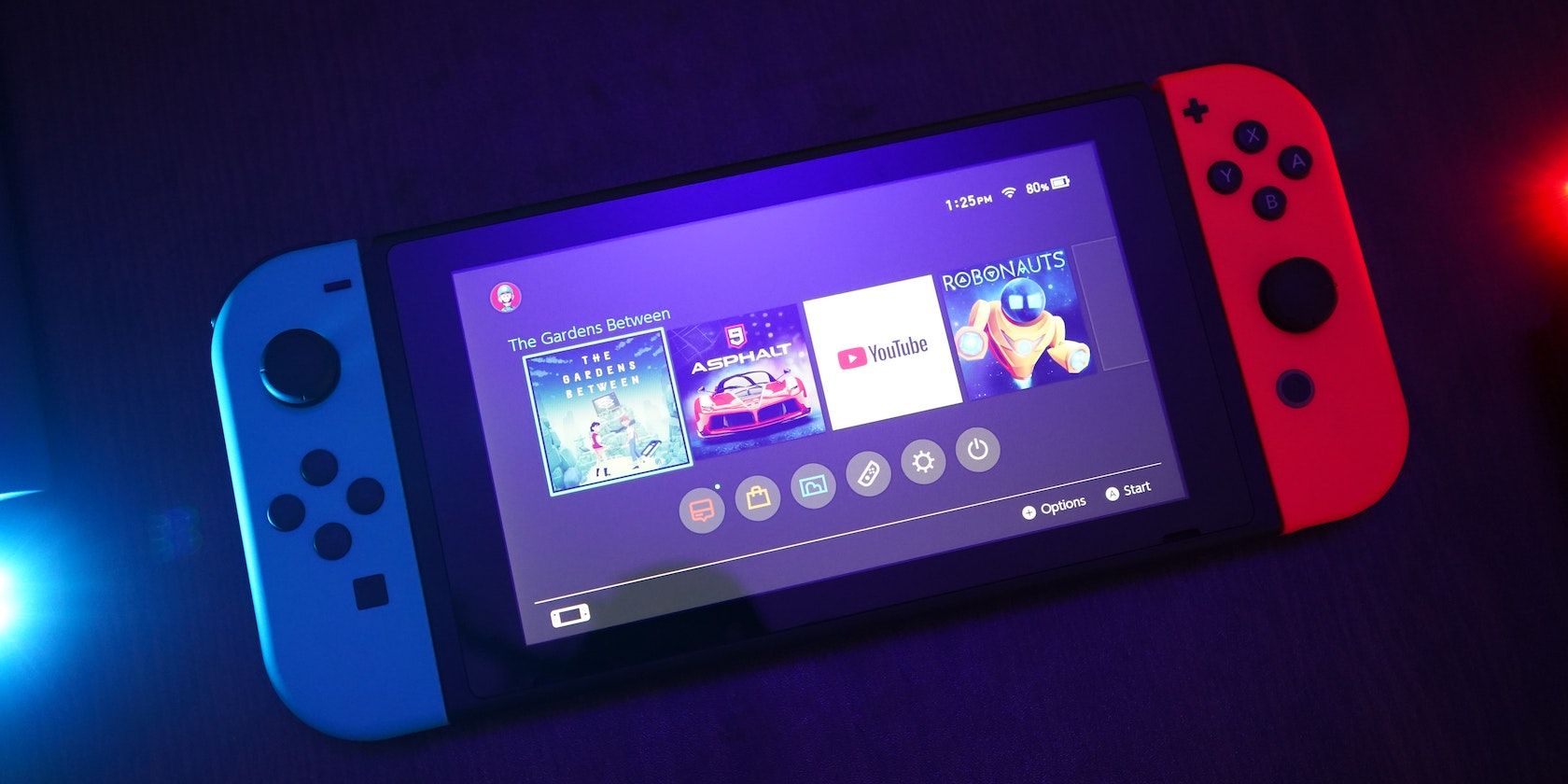This detailed image appears to be a close-up photograph of a Nintendo Switch, a portable gaming console known for its distinctive design and vibrant colors. The device has a blue border on the left side and a red border on the right side, with its signature large black control knobs on either side of the screen. The rectangular screen in the center displays a game selection interface with a purple background, featuring four distinct tiles: one with an image resembling a car, another with the YouTube logo against a white background, a third displaying what appears to be an alien creature, and a final tile that looks like the front cover of a video game, possibly titled "The Gardens Between." The overall photograph has a dark blue and dark purple blurry background with gradients created by blue and red orbs, adding to the contemporary and dynamic feel of the scene.